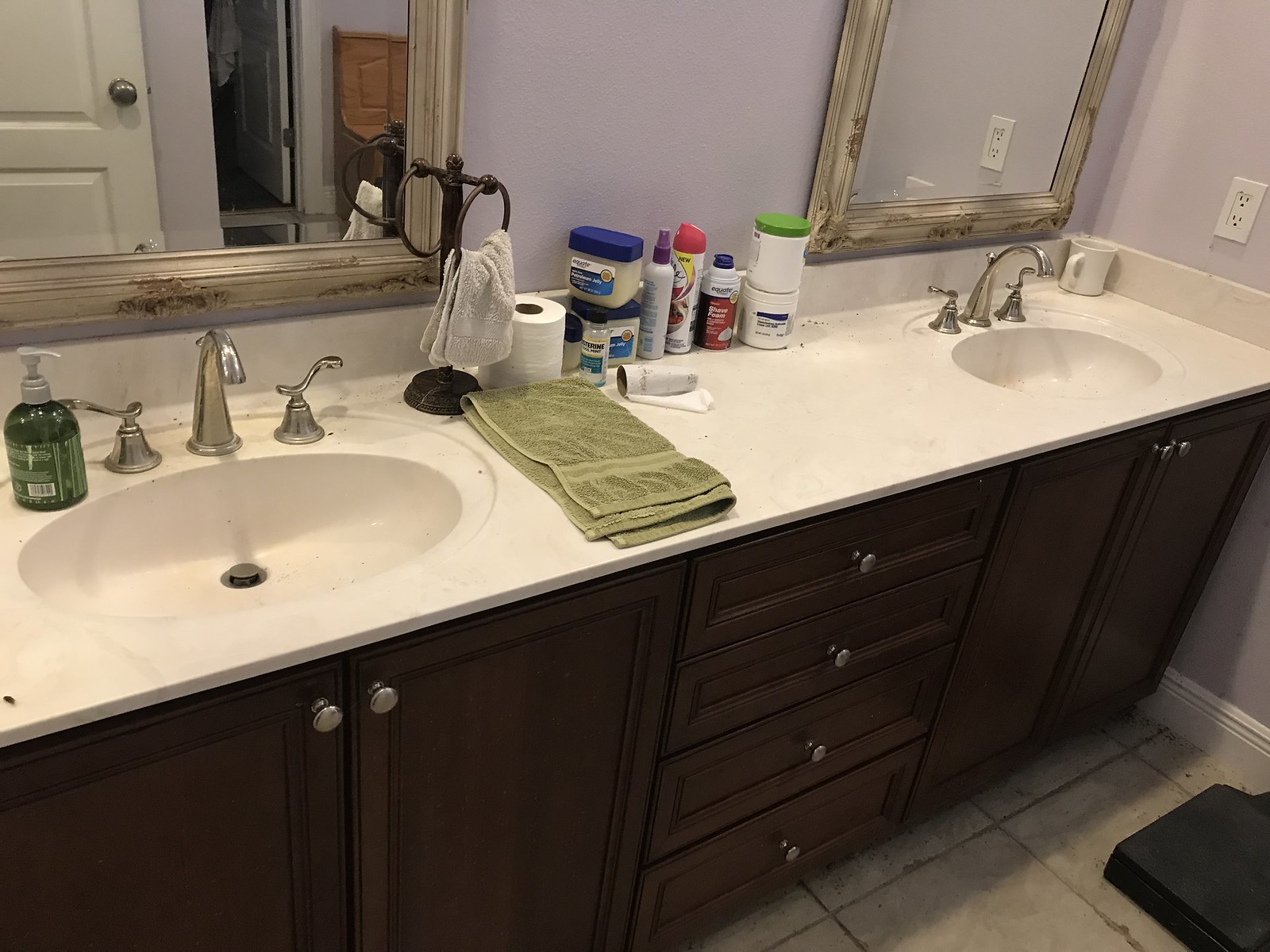The photograph showcases a meticulously arranged double-sink bathroom. The focal point of the image is the expansive, off-white countertop that houses two integrated sinks. Each sink features metal fixtures with distinct handles for hot and cold water. Between the two sinks, a variety of personal care products, including bottles and jars of ointments and shaving cream, are neatly organized. A roll of toilet paper is positioned to the left of this collection.

Above each sink, a wooden-framed mirror reflects the light, adding depth to the room. The walls are painted a soft, light purple, accented by a crisp white molding at the base. The floor is covered in dark brown or brown-gray tiles that contrast elegantly with the light walls.

Below the countertop, the cabinets are crafted from dark wood, adding a touch of sophistication. Each sink is flanked by two cabinet doors, while four additional drawers are situated between the sinks, offering ample storage space. A neatly folded green towel is placed at the edge of the countertop, centrally located between the two sinks, adding a subtle pop of color to the overall neutral palette of the bathroom.